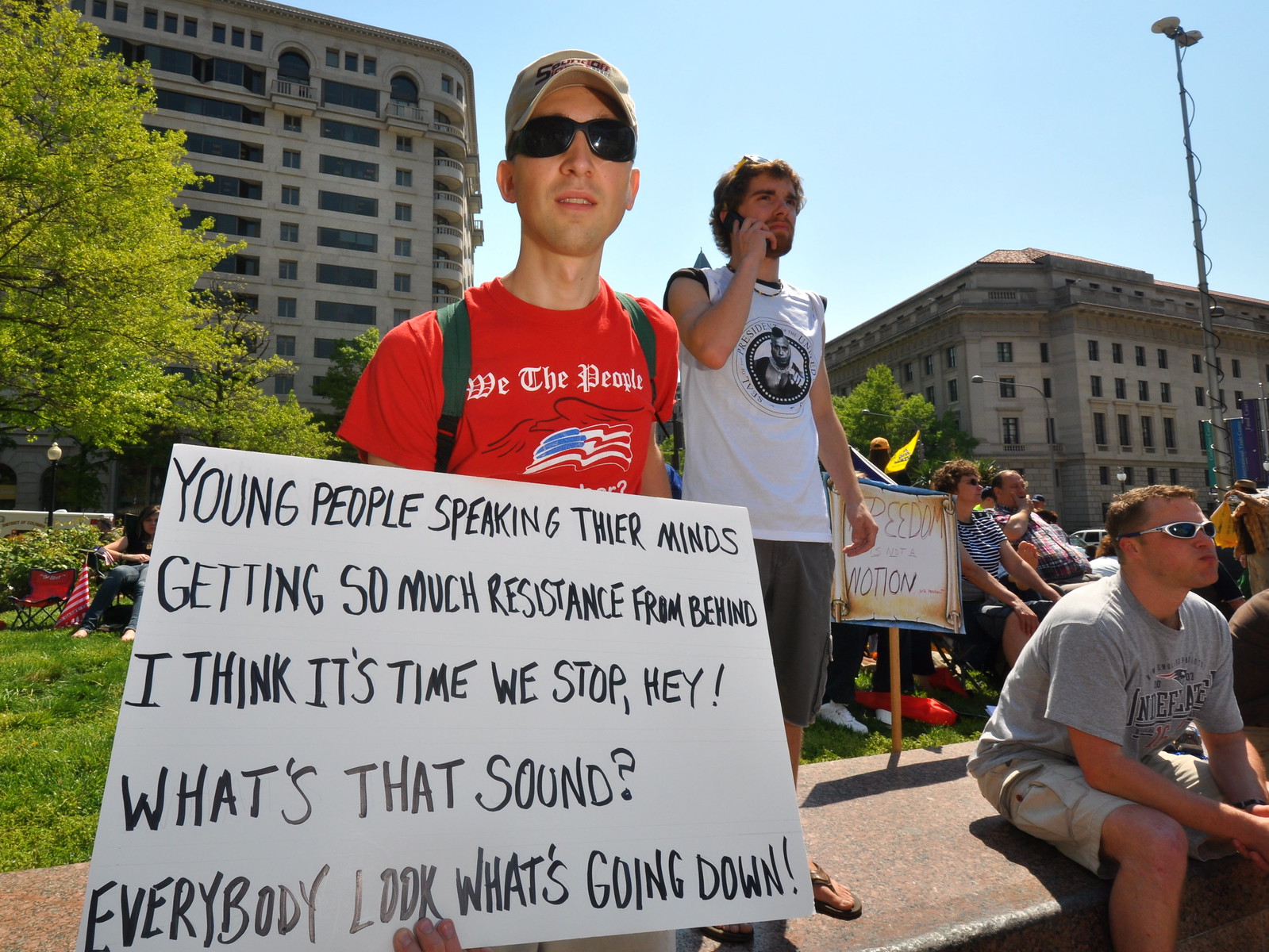The image depicts an outdoor political event, possibly a protest or rally, taking place on a warm day. The setting features a mix of college-age attendees and older individuals, with a noticeable focus on younger people. In the foreground stands a young man wearing a red shirt with the inscription, "We the People," along with a baseball cap and black sunglasses. He holds a poster board that reads: "Young people speaking their minds, getting so much resistance from behind. I think it's time we stop. Hey, what's that sound? Everybody look, what's going down?"

The attendees are gathered on a grassy knoll area, with some seated on folding chairs, indicating they might be listening to a speaker. The backdrop includes tall buildings, which appear to be apartments or hotels, and a broadcasting truck with a telescoping light tower. A few trees dot the landscape, enhancing the outdoor setting. Additionally, visible signs include one resembling a scroll with the message "Freedom is not a notion" and a Gadsden flag, suggesting the event may lean towards libertarian or conservative viewpoints.